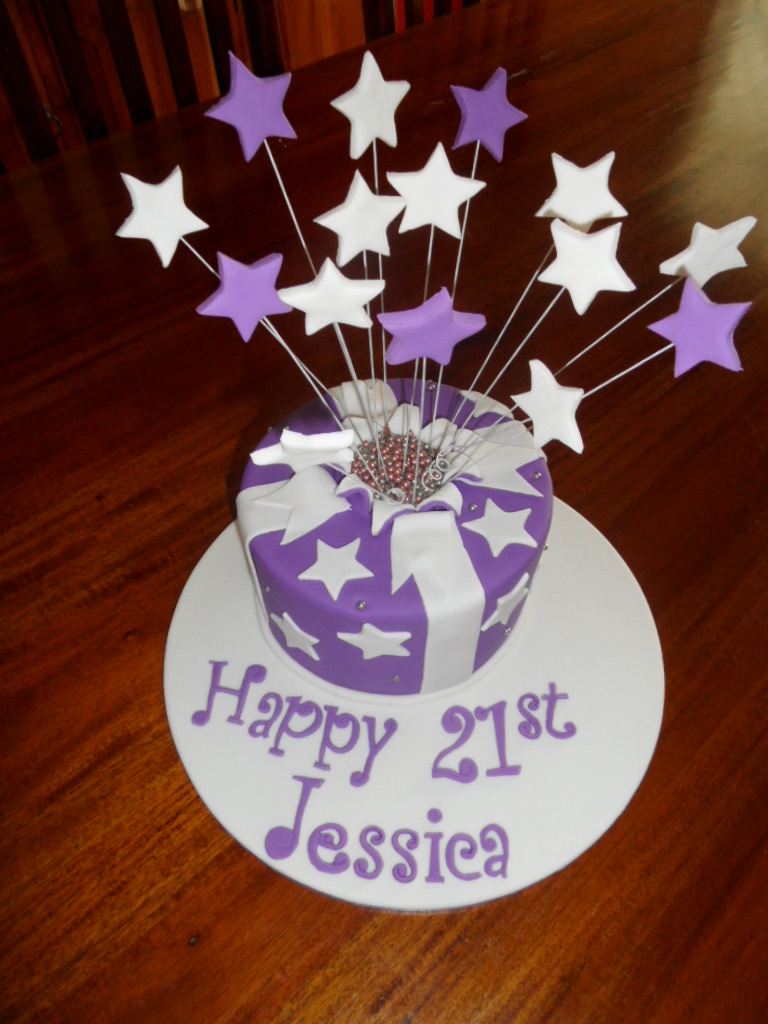The image depicts a richly colored wooden table, reminiscent of redwood or mahogany, accompanied by matching wooden chairs. Atop the table sits a circular white plate holding a festive birthday cake. The cake, primarily purple with white star embellishments, is adorned with an elegant white frosting ribbon that wraps up the sides and forms a bow at the center. This central bow is decorated with small beads, from which about a dozen sticks extend, each topped with either a white or purple star, resembling a burst of celebratory fireworks. Positioned slightly off-center on the plate, the cake bears the inscription, "Happy 21st, Jessica," in playful purple writing, completing the joyful scene.